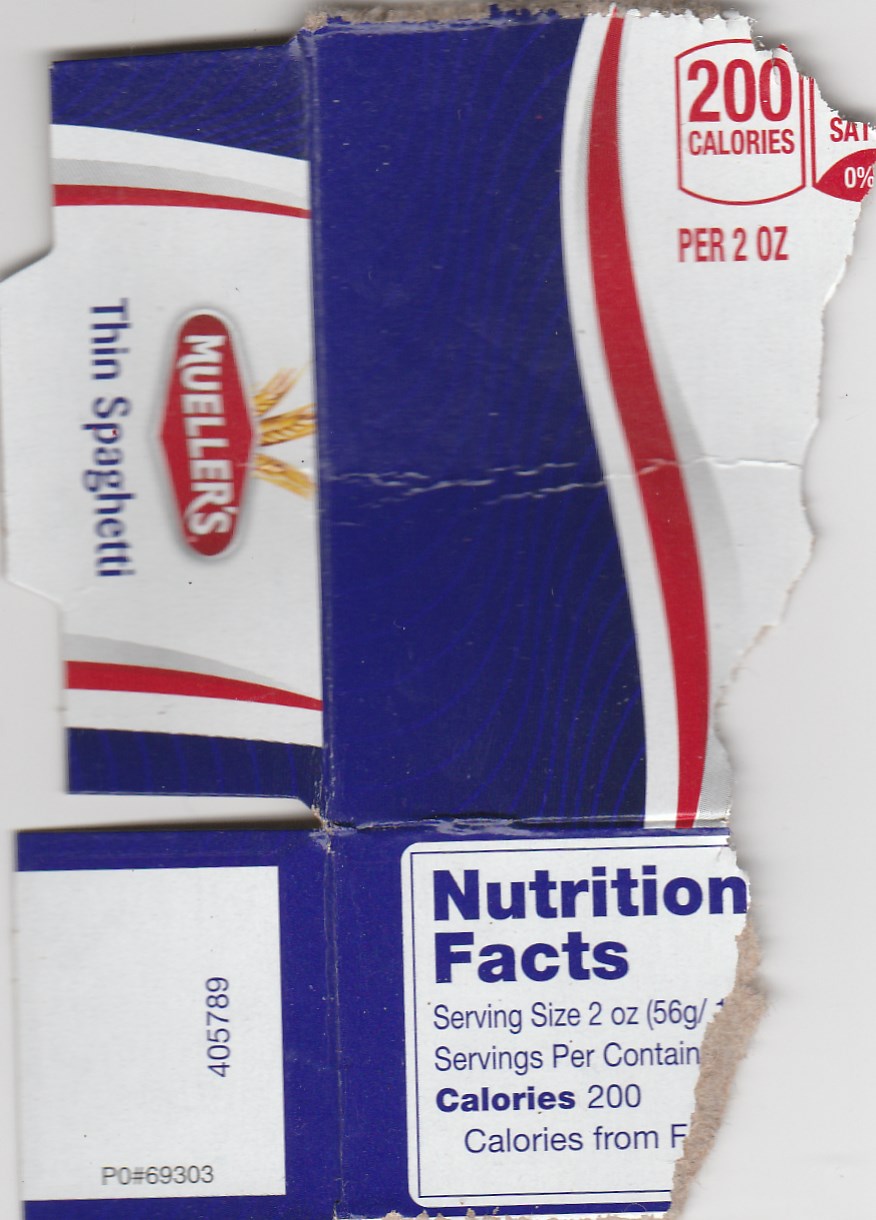The image depicts a partial, torn piece of a cardboard box of Mueller's Thin Spaghetti against a white background. The box features a familiar red, white, and blue color scheme, with a predominantly blue top and sides, a large white section in the middle, and a red stripe along the side. The Mueller's logo, with three wheat stalks emerging from the top, is visible in white letters on a red sign in the middle of the box. Below the logo, the product name "Thin Spaghetti" is printed in blue letters. The top-right corner prominently states "200 calories per two ounces" in red letters. The Nutrition Facts panel, partially torn, is shown in blue font, indicating a serving size of 2 ounces and 200 calories per serving. Additionally, part of the manufacturing lot codes is visible in the bottom corner of the image.